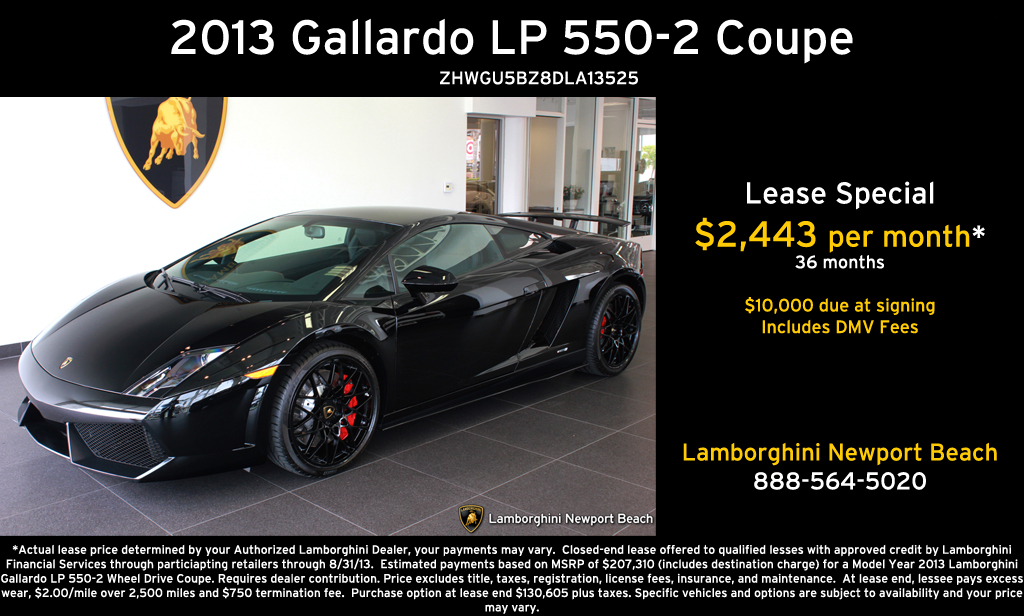This advertisement features a striking black Lamborghini Gallardo LP 550-2 Coupé from 2013. The top of the image prominently displays the car model's name, followed by the VIN ZHWGU5BZ8DLA13525. Below, the black Lamborghini, which boasts black wheels with red accents, is showcased in a tiled garage. On the white wall beside the car, there is a Lamborghini logo shield with a gold bull. The leasing details to the right of the image state a lease special of $2,443 per month for 36 months with $10,000 due at signing, which includes DMV fees. The dealership information, Lamborghini Newport Beach, is also provided along with the contact number 888-564-5020. The bottom of the image contains additional fine print terms for leasing.